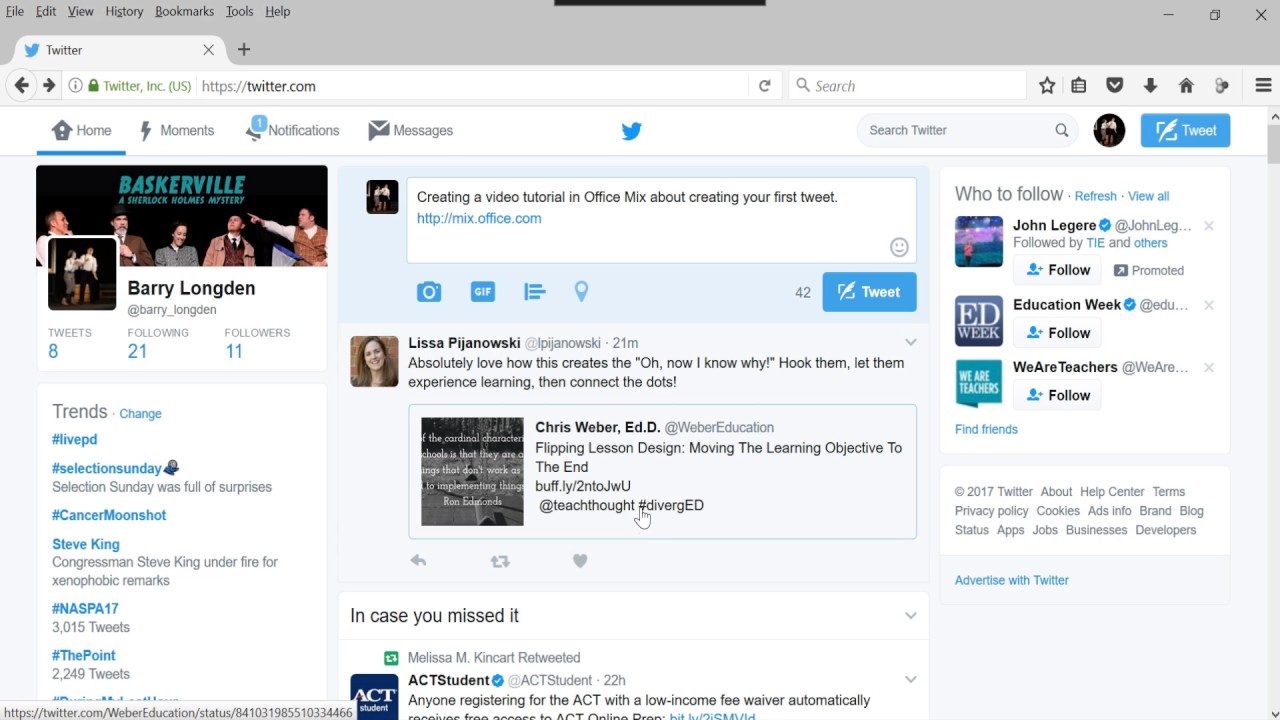The image showcases a Twitter webpage featuring a user profile and various interface elements. In the top left corner, the Twitter logo and URL (twitter.com) are displayed. The left sidebar contains navigation options: Home, Moments, Notifications (showing one notification), and Messages, followed by the active blue Twitter bird icon.

Below these tabs, the user profile section reads "Baskerville: A Sherlock Homeless Mystery," attributed to Barry Longden (@Barry_Longden), who has 8 tweets, follows 21 accounts, and has 11 followers—the numbers for these stats are highlighted in blue.

At the bottom left of the page, trending topics are listed: #LiveBD, #SelectionSunday, #CancerMoonshot, #SteveKing, #NASPAS17, and #DPoint. On the right side, there is a status update box titled, "Create a video tutorial in Office Mix about creating your first tweet." The 'Tweet' button is located within this box, accompanied by icons for adding a camera, GIF, poll, and location.

A recent tweet from Lisa Pijanowski (@LPijanowski), posted 21 minutes ago, reads: "Absolutely love how this creates the 'Oh, now I know! I hope to let them experience learning, then connect the dots.'" Below it, in the "In case you missed it" section, a retweet from Medics & King Cut from a City student states: "Anyone registering for the A City with a low income will automatically receive free access to A City Online Prep."

The right side also features a "Who to follow" suggestion list with a "Refresh" option and a "View all" link, showcasing users like John Legere, Education Week, Days, and We Are Teachers.